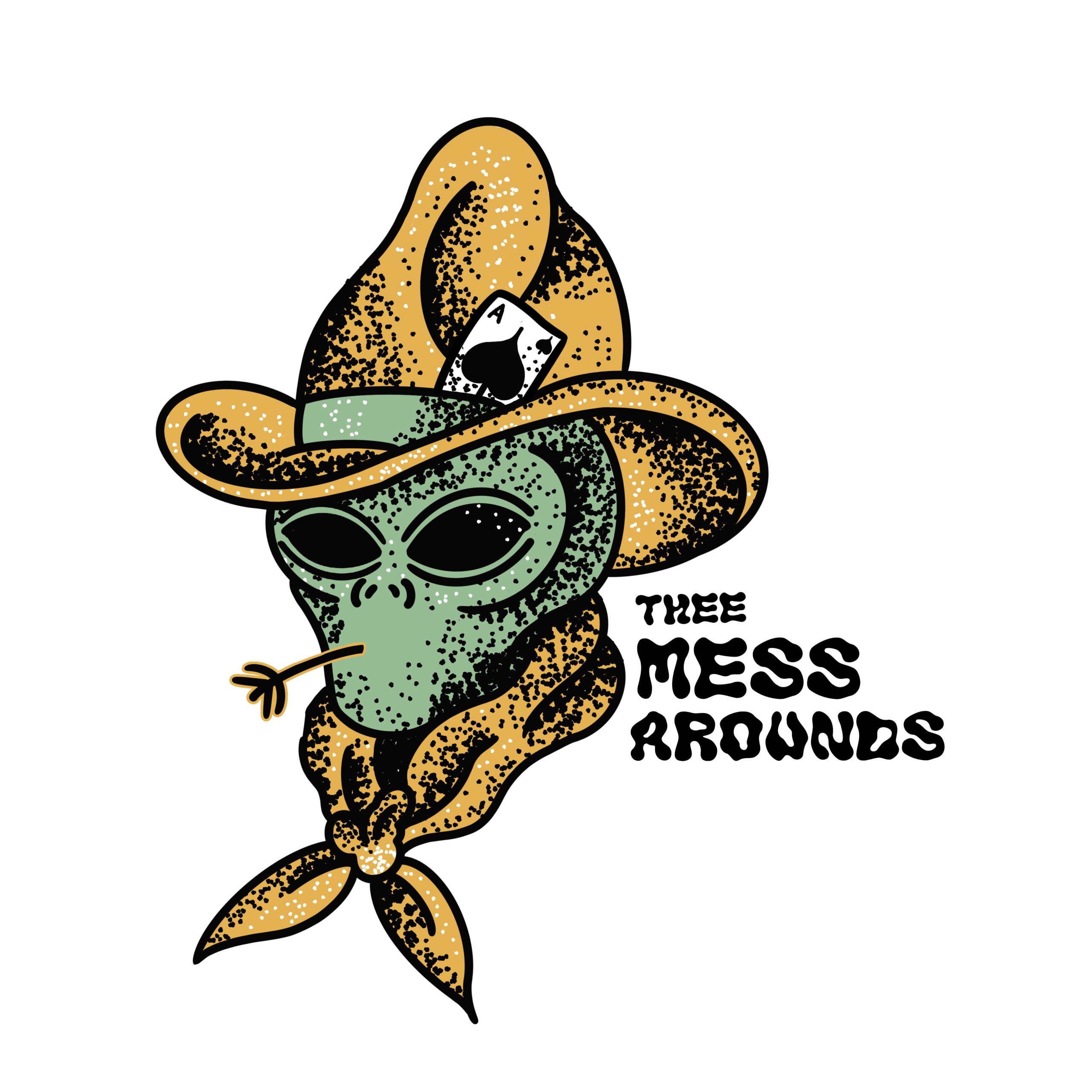The image features a stylized, cartoonish alien with a green face and large, black, horizontally elongated eyes, exuding a distinct Old West vibe. The alien is adorned with a brown-rimmed cowboy hat, complete with a green ribbon around the brim where a white ace of spades playing card, outlined in black, is tucked in. The card has a prominent black spade and an 'A' in the upper left corner. Below the hat, a brown scarf is tied neatly around the alien's neck in a bow. The alien's face, along with the hat and scarf, is speckled with black dots, enhancing the graphic's texture. Interestingly, a yellow straw with a black outline extends from the mouth area, adding to the Western theme. The background is a clean, stark white with no borders, emphasizing the central character. To the right of the alien, in a squiggly, alien-like font, the text "He Mess Arounds" is prominently displayed, suggesting a possible band name or album title. Overall, the detailed elements and unique styling give the impression of a creative and possibly musical theme.